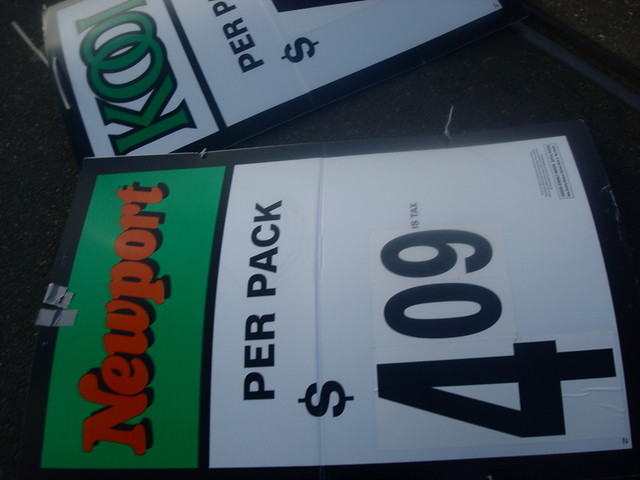In this landscape-oriented photograph, rotated 270 degrees to the right, we observe a dimly lit scene featuring price tags for cigarettes. Dominating the bottom portion of the image is a price tag with a distinctive green header displaying the brand name "Newport" in bold red text. Just beneath, in black text, it reads "per pack," followed by the price "$4.09," with an additional note mentioning tax, though it’s unclear if the price is inclusive or exclusive of tax. Above this tag, there is another price tag with "Kool" written in green text. However, the remaining details of the Kool price tag are cut off and not fully visible. The overall ambiance of the photo is quite dark, and the rotated perspective adds a unique and slightly disorienting view of the cigarette price tags.